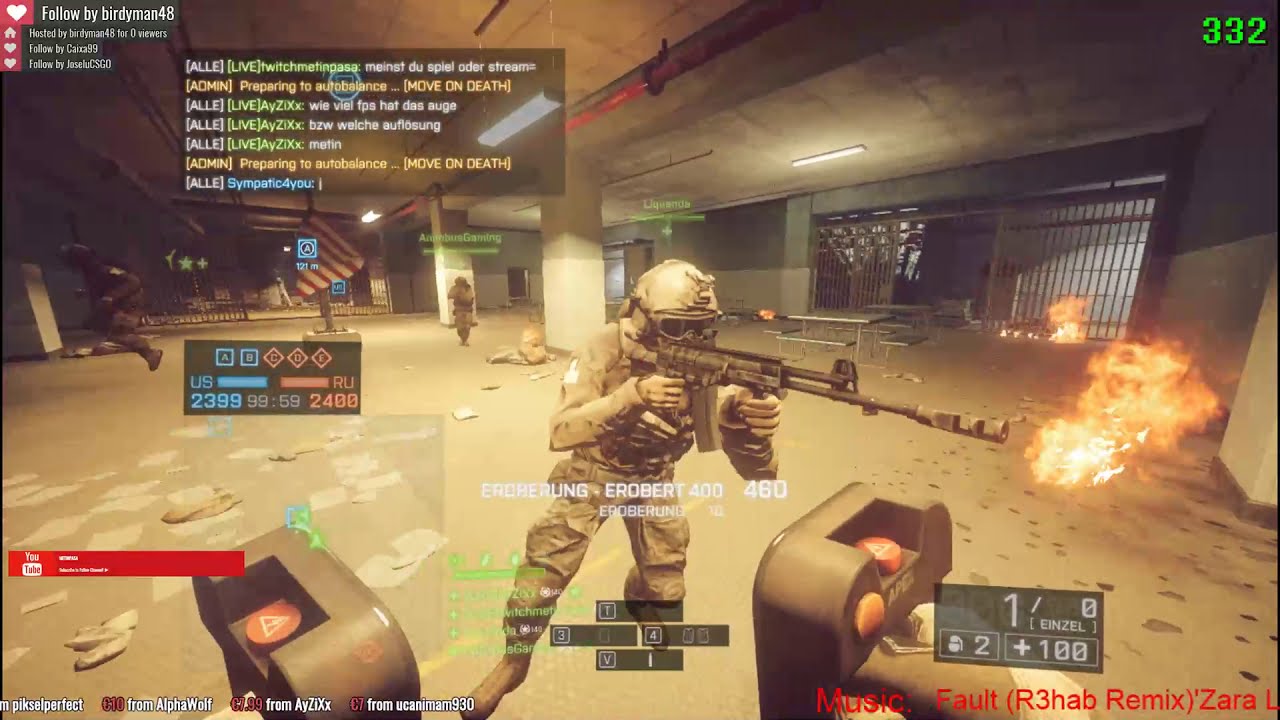This image is a detailed screenshot from a first-person shooter game. At the center stands a soldier clad in camouflage and a helmet, gripping a long rifle with an extended ammo clip. His right hand holds the handle at the rear of the rifle, while his left hand supports the front. The rifle is angled slightly downwards to the right. The floor beneath him is a sandy yellow color, suggestive of a warehouse or commercial building setting, with patches of fire visible on the ground.

Icons and texts populate the screen, adding layers of informational overlays. In the upper-left corner, a heart icon accompanies the text "follow by Birdman 48," coupled with additional icons and white text mentioning hosting details. A chat box dominates part of the screen with names like Allie and Admin exchanging messages, including foreign language text and instructions like "prepare to auto balance, move on death."

In the top-right corner, the number 332 is displayed in green. Meanwhile, on the bottom-right, red text reads "music fault (R3HAB remix)," followed by "ZARA L."

The scene also depicts other players in military gear, with some moving in the background and a teammate holding what appears to be a defibrillator. In the distance, a significant gate structure is visible, reinforcing the setting's warehouse-like atmosphere.